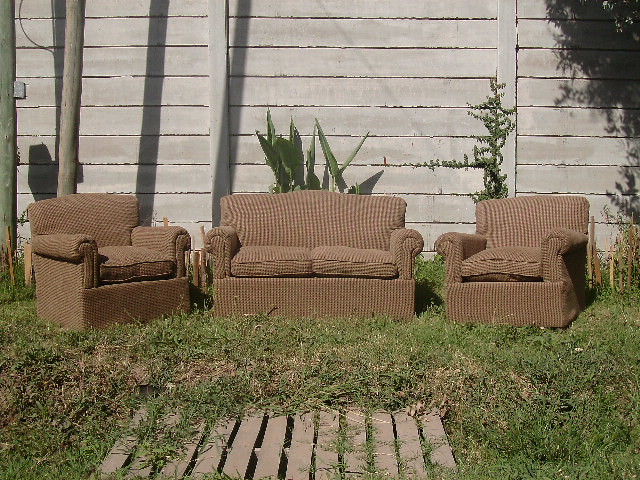The photograph captures an outdoor scene set against the side of a weathered, wooden barn characterized by horizontal boards. In the foreground, there is an arrangement of three pieces of cushioned furniture resembling a living room set placed on untamed, grassy terrain. This set includes a loveseat with two cushions and armrests situated in the middle, flanked by two matching single-seater chairs on either side. All the furniture shares a burgundy or light brown checked pattern with dark brown stripes and appears to be designed for comfort, featuring soft cushions and rolled arms.

Directly in front of the seating arrangement, a wooden pallet or grate lies partially buried in the grass, with blades growing through its slats, indicating it has been there for a while. Surrounding the furniture are various plants, including some green, spiky-leaved plants and a vine climbing the barn's grayish wooden fence. Additionally, a tall dark green plant, possibly a cactus, and the shadow of a tree are visible near the furniture. The scene is consistent with a rustic yet cozy backyard setting, emphasized by the aged, bleached appearance of the wooden details and the natural overgrowth.